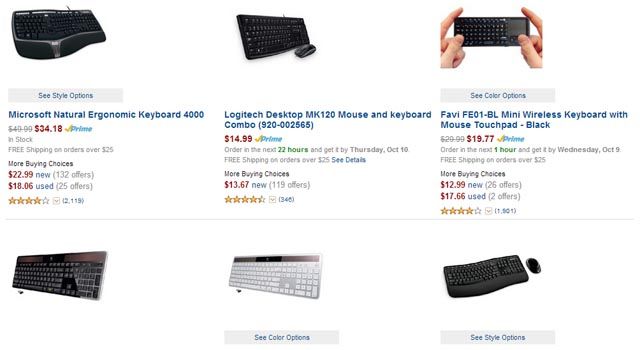**Detailed Caption for Image:**

The image features six different product listings, each displayed with detailed information including name, price, purchasing options, and customer ratings. 

1. **Microsoft Natural Ergonomic Keyboard 4000**:
   - Displayed with a blue name banner against a gray background.
   - **Price**: $34.18 (discounted from $49.99).
   - **Amazon Prime**: Free shipping on orders over $25.
   - **More Buying Choices**: Available for $22.99 (new) and $18.06 (used).
   - **Customer Ratings**: 4 stars from 2,119 reviews.
   
2. **Logitech Desktop MK120 Mouse and Keyboard Combo**:
   - Blue name banner with precise listing details.
   - **Price**: $14.99.
   - **Amazon Prime**: Order within the next 22 hours for availability.
   - **More Buying Choices**: Available for $13.67 (19 offers in total).
   - **Customer Ratings**: 4 gold stars.

3. **Fabay FE01BL Mini Wireless Keyboard with Mouse Touchpad, Black**:
   - Blue name banner with all specifications.
   - **Price**: $19.77 (original price $29.99).
   - **Amazon Prime**.
   - **More Buying Choices**: Available for $12.99 (new) and $17.66 (used).
   - **Customer Ratings**: 4 gold stars from 1,801 reviews.
   
4. **Visual Summary of Remaining Keyboards**:
   - Three additional black keyboards are depicted above the text-based listings.
   - One keyboard in the middle is silver, with a note "see color options".
   - The rightmost black keyboard mentions "see style options" but lacks further description.

Additionally, all products have clear Prime checkmarks in blue, indicating their availability for Amazon Prime services. Each listing is structured with prices in red, customer star ratings in gold, and the name of the products consistently highlighted in blue.